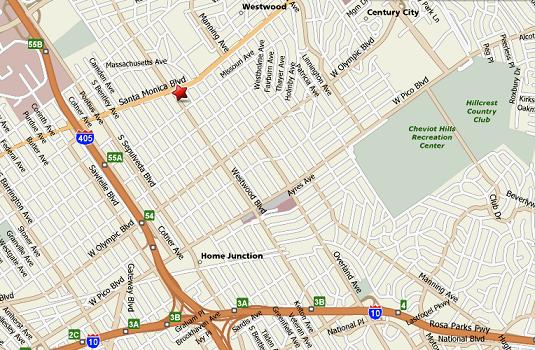This image depicts a map resembling the traditional paper maps commonly found at gas stations. Unlike the typical digital interface of Google Maps, this map showcases streets in varying shades of light to dark orange. The current location appears to be indicated by a prominent red star situated at the top left corner, positioned just below Santa Monica Boulevard on Massachusetts Avenue, and pointing towards the bottom right of the image.

The streets are labeled with green and white, as well as blue and white text. For instance, a green and white street sign identifying "55B" is visible at the top left of the map. Additional landmarks and areas of interest are marked, such as Century City at the top right, the Chevrolet Hills Recreation Center, and the Hillcrest Country Club positioned below Century City.

While the red star likely signifies either the current location or a destination, the map does not provide specific directionality or navigational intent, leaving the exact purpose somewhat ambiguous.